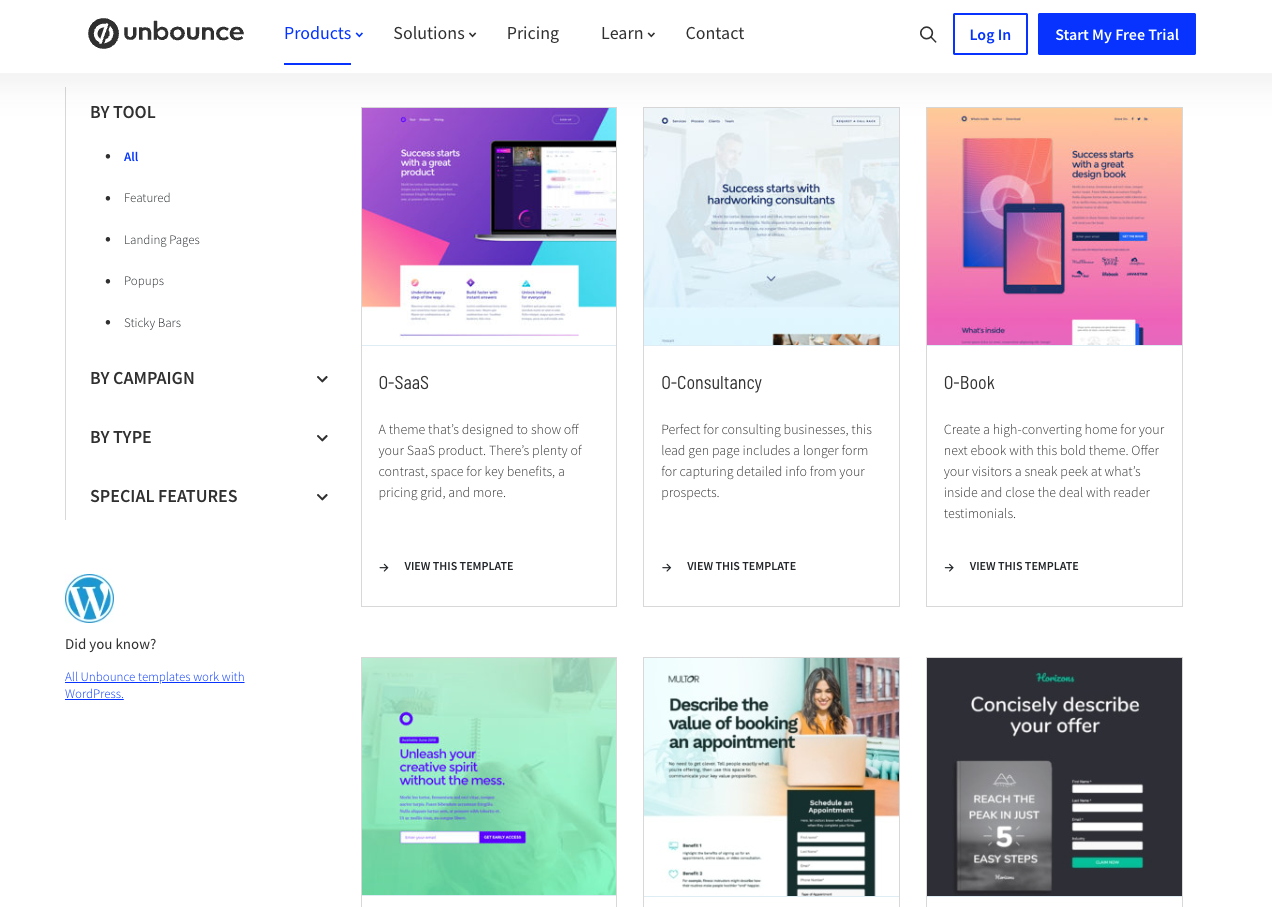The homepage of the Unbounce website prominently displays their logo in the top left corner. The logo features a circular design with a protractor-like shape and a half-circle arc in white text, set against a black circle, accompanied by the company name "Unbounce" in black text.

At the top of the landing page, a navigation bar provides links to "Products," "Solutions," "Pricing," "Learn," and "Contact," as well as options to search, log in, and start a free trial, indicative of a product offering.

On the left sidebar, there are categorical options labeled by tool: "All Landing Pages," "Pop-Ups," "Sticky Bars," and an unreadable fourth option. Additionally, there are dropdown menus under "Campaign," "Type," and "Special Features" for further navigation.

The main section of the page is organized with various rectangular blocks showcasing different templates. The first row includes templates named "0-SAAS," "0-Consultancy," and "0-Book," each accompanied by a short description and a "View This Template" button, suggesting that clicking on these will display the respective template.

Below this, three more template options are displayed:
1. "Unleash Your Creative Spirit Without the Mess."
2. "Describe the Value of Booking an Appointment."
3. "Concisely Describe Your Author."

These sections provide further template options for various business needs, allowing users to preview and select templates that suit their requirements.